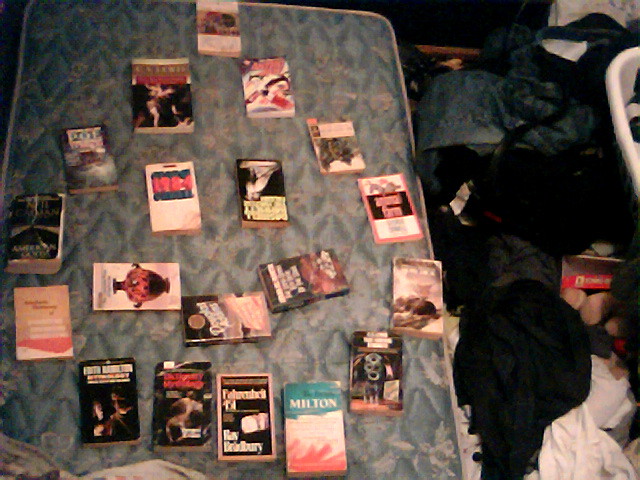This color photograph, taken from above, captures a cluttered and untidy bedroom. At the center is a bare, blue mattress with no sheets or covers, prominently displaying a collection of various paperback books and VHS movies. The titles of the media are somewhat legible, with mentions of "1984" and "Fahrenheit 9-11" seen among the books, while a VHS tape labeled "Milton" is also visible. The mattress supports at least 18 different items, including books, whose covers are mostly aged and a bit blurry, and possibly written in different languages, including one that might be German.

The surrounding room is in disarray, with heaps of clothes strewn across the floor. There is a noticeable presence of a white laundry basket peeking from the right edge of the image. Among the scattered clothing, a blue shirt can be identified. The overall indoor lighting is dim, adding to the chaotic and cluttered feel of the space.